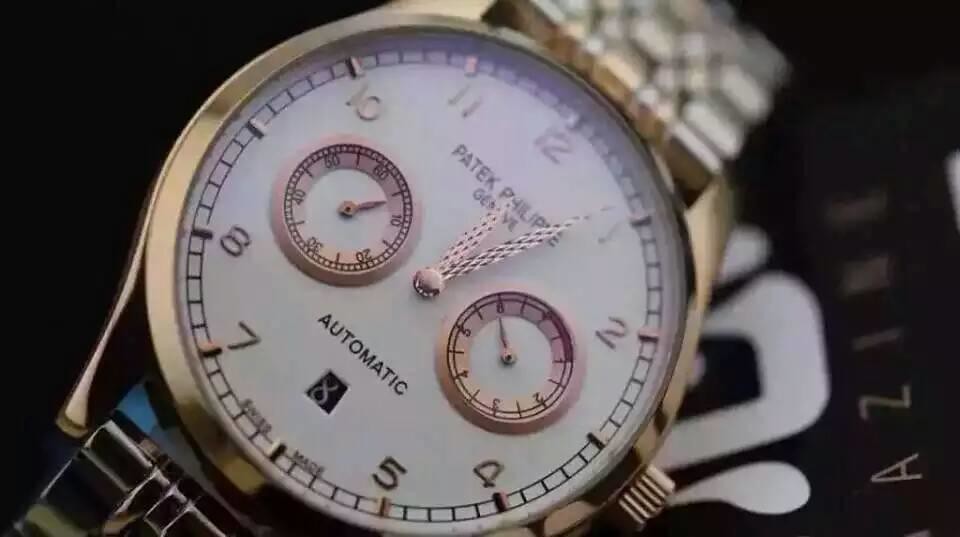This rectangular photograph, oriented horizontally, showcases a sophisticated men's automatic watch from the prestigious brand Patek Philippe, Geneva. The watch's elegant design features a predominantly white face, encased in a luxurious gold frame with a gold and silver bracelet. Delicately crafted gold hands, with the hour hand pointing towards 12 and the minute hand at the 4-minute mark, stand out against the watch's face.

The watch features raised gold numerals, excluding the 3, 6, and 9, and minute markers encircling the dial. Notably, the face includes two smaller rose gold-toned sub-dials; one possibly a directional compass, while the other likely functions as a seconds counter marked from 10 to 60. The text "Patek Philippe" and "Geneva" is prominently displayed in black above the center of the face, with "Automatic" inscribed just above a small window at the bottom. The watch stands out against a black background, further emphasizing its luxury and precision.